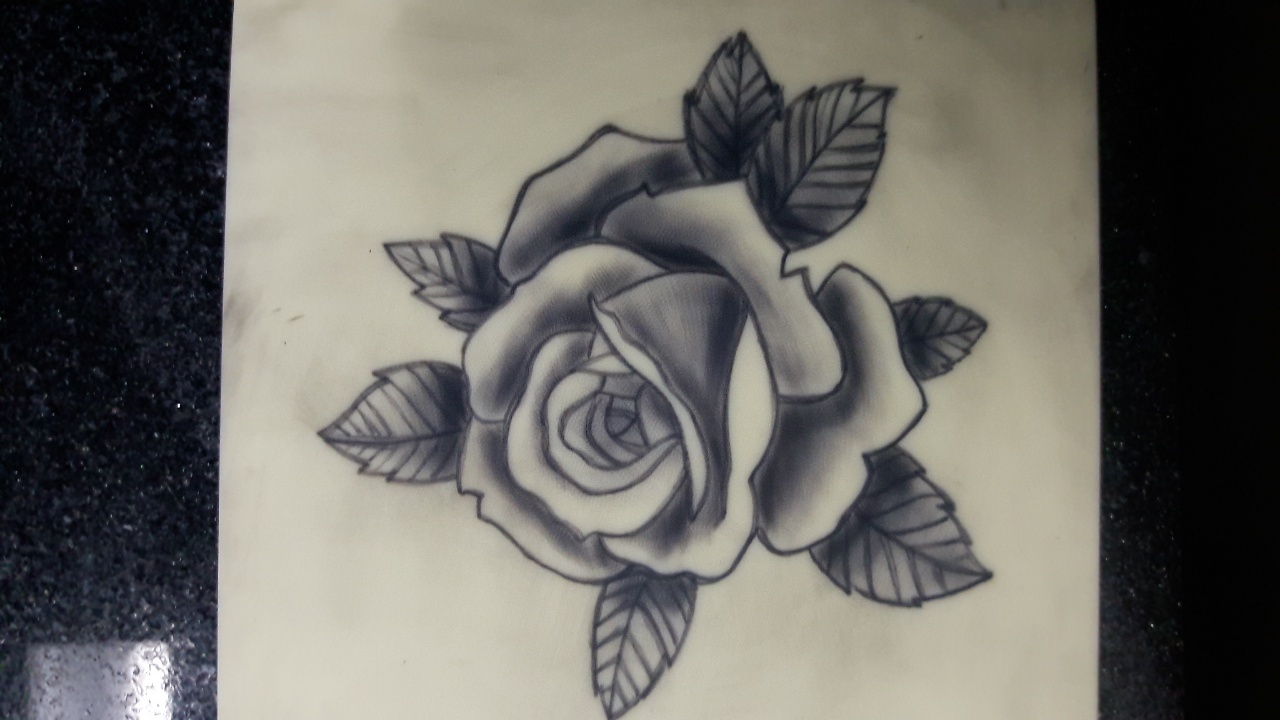The image showcases a detailed drawing of a rose, set on a black marble table with specks. The central focus is a nearly fully bloomed rose, sketched in monochrome, with varying shades created by pencil, charcoal, or ink. The drawing rests on a piece of paper that appears grey and mottled, possibly smeared with ink. Positioned close to the center of the paper, the rose is slightly tilted downwards to the left, revealing its intricate inner petals and multiple layers. Surrounding the rose are seven leaves, differing in size and direction: some stretch upward and to the side, while others extend downward. The image likely captures natural and artificial light reflections, suggesting it was taken in daylight. A hint of glitter adorns the bottom left corner of the marble surface.